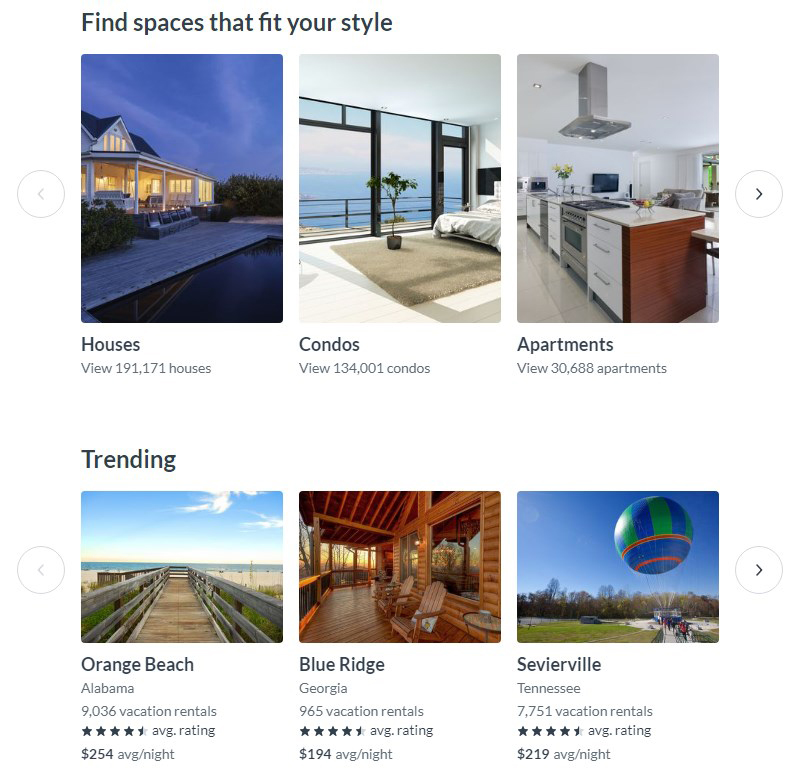The top left of the image features the text "Find spaces that fit your style" set against a white background. There are six smaller images displayed, each showcasing different types of living spaces with accompanying text and statistics.

- The first image, located on the top left, is labeled "Houses." It invites viewers to explore "191,171 houses" and features a white house with a black roof. The house is illuminated with yellow light, set against a clear blue sky. A swimming pool in the foreground reflects the sky, adding to the serene ambiance.
  
- The second image is labeled "Condos." Viewers are prompted to "view 134,001 condos." The picture shows the interior of a condo with a white bed and brown carpets. A large window offers a stunning ocean view, complemented by a green potted plant.

- The third image is dedicated to "Apartments" and encourages viewers to "view 3,388 apartments." The image depicts a modern kitchen with grey appliances and a mix of white and brown tables.

Transitioning to the bottom row, there are three images under the label "Trending."

- The fourth image, in the bottom left, focuses on "Orange Beach, Alabama." It highlights "9,036 vacation rentals" with an average rating of 4.5 stars and an average price of $254 per night. The picture shows a picturesque beach scene.

- The fifth image in the center showcases "Blue Ridge, Georgia." It mentions "6,965 vacation rentals" with a 4.5-star rating and an average cost of $194 per night. The image features a scenic view representative of the Blue Ridge area.

- The sixth and final image, located on the bottom right, features "Sevierville, Tennessee." It details "7,751 vacation rentals" with a 4.5-star rating and an average nightly price of $219. The image captures a typical vacation rental scene in Sevierville.

Together, the collection of images and their detailed descriptions provide a comprehensive overview of various rental options, each catering to different preferences and styles.